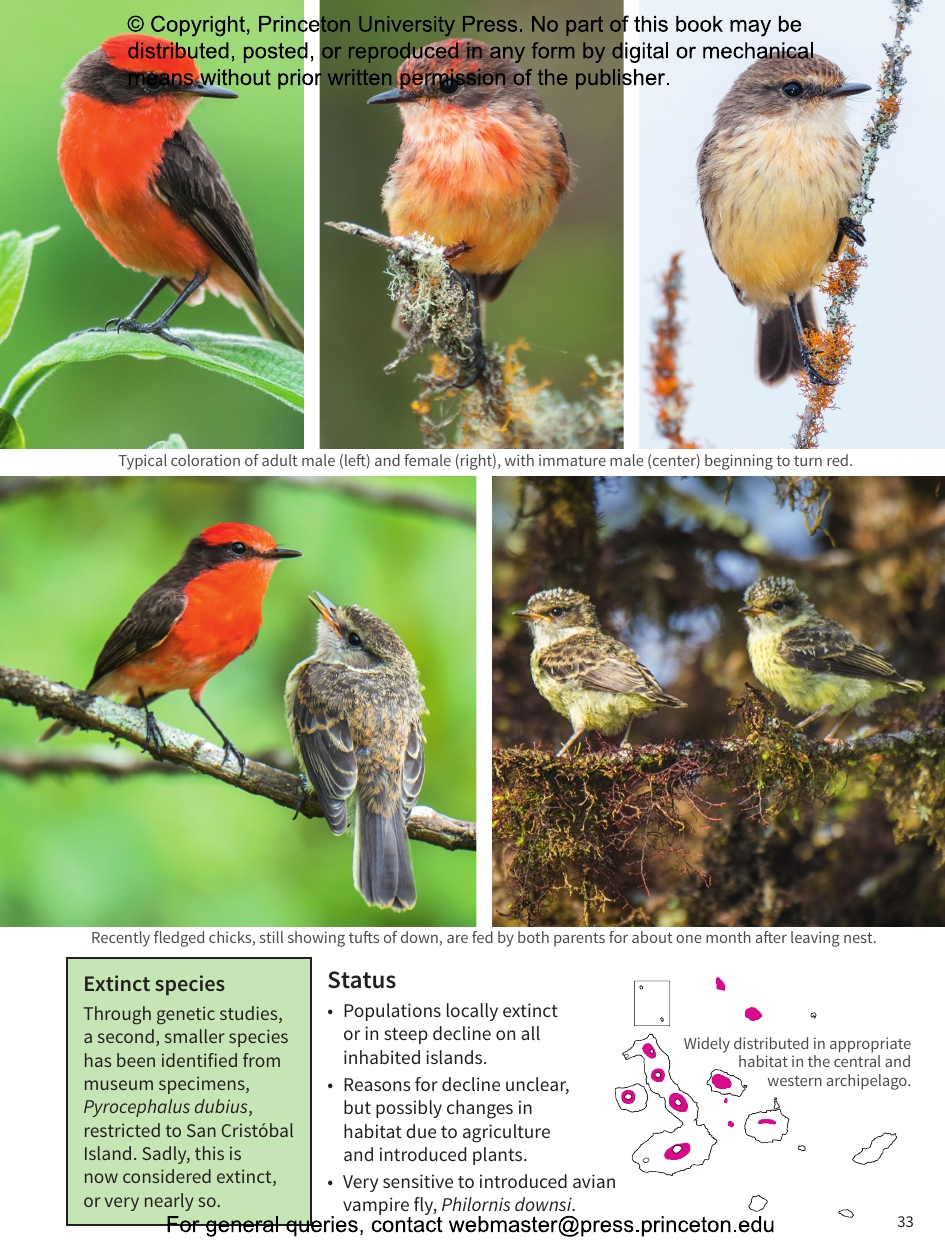The image is of a page from a bird textbook, published by Princeton University Press, as indicated by the copyright notice at the top. The page features five color photographs of small songbirds, along with explanatory text. 

At the upper left, a small bird with a red body, black wing, and a black stripe over its eye perches on a plant. To its right, another small peach-colored bird with a black beak and eye sits against a moss green background. Next, on a white background, a bird clutching a branch is depicted with a yellow breast, brown head, black beak, and black feet. The text above these images states: "Typical coloration of the adult male (left), the female (right), and an immature male (center) beginning to turn red."

Below these images, a photo shows two birds on a branch with a green background: one bird resembles the bright red male from the first photo, while the other has similar shape and features but with dark brown feathers. Next to this image, another photo shows two young birds with yellow breasts, brown wings, and brown heads, seemingly recently fledged chicks with tufts of down. The accompanying text reads: "Recently fledged chicks still showing tufts of down are fed by both parents for about one month after leaving the nest."

At the bottom of the page, a green text box describes the status of an extinct species, Pyrocephalus dubious, once restricted to San Cristobal Island and now considered extinct or nearly so. It notes the species' decline due to habitat changes from agriculture and introduced plants, as well as sensitivity to the introduced avian vampire fly, Philornis downsi. To the bottom right is a line drawing of a map with pink dots on land masses, indicating the distribution in the central and western archipelago.